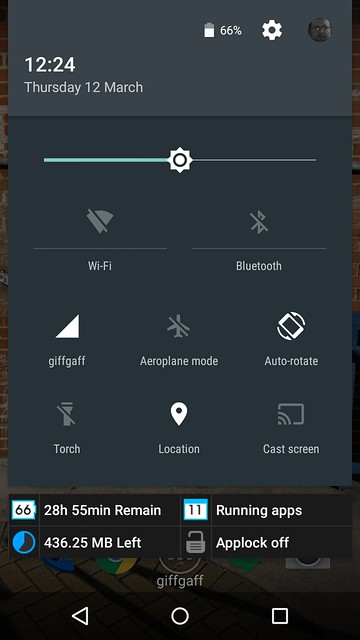### Detailed Caption

The image displays a smartphone interface highlighting various informational and functional elements on the screen. At the very top center, there is a digital clock displaying "12:24" in bold white text. Directly underneath, in a lighter font, it reads "Thursday, 12 March." The top right corner contains a battery icon indicating 66% charge remaining, alongside a small gear icon for accessing settings. Next to the gear is a profile picture placeholder symbolizing the user's avatar.

Below this section lies a brightness adjustment slider, currently positioned at the midpoint. Further down, there are indicators for Wi-Fi and Bluetooth connectivity, followed by two rows of three functional icons each. The first row contains, from left to right: 
1. A "GIF GAF" icon represented by a right-facing triangle.
2. An airplane mode icon.
3. An auto-rotate icon depicted by a rotating phone.

The second row features:
1. A torch icon with a flashlight symbol struck through by a line, indicating the flashlight is off.
2. A location icon.
3. A cast screen icon.

Among these icons, "GIF GAF," auto-rotate, and location are highlighted, indicating they are active functions.

Further down the screen, text displays "28 hours 55 minutes remain," alongside a box stating "66" and another box displaying "11," indicating there are 11 running apps. Below this, additional information reads "Time left: 436.25 MB," followed by an "App Lock: Off" status.

At the bottom of the screen, three navigation icons are visible:
1. A back arrow to the left.
2. A circle in the middle, likely for returning to the home screen.
3. A square on the right, probably to view recent apps.